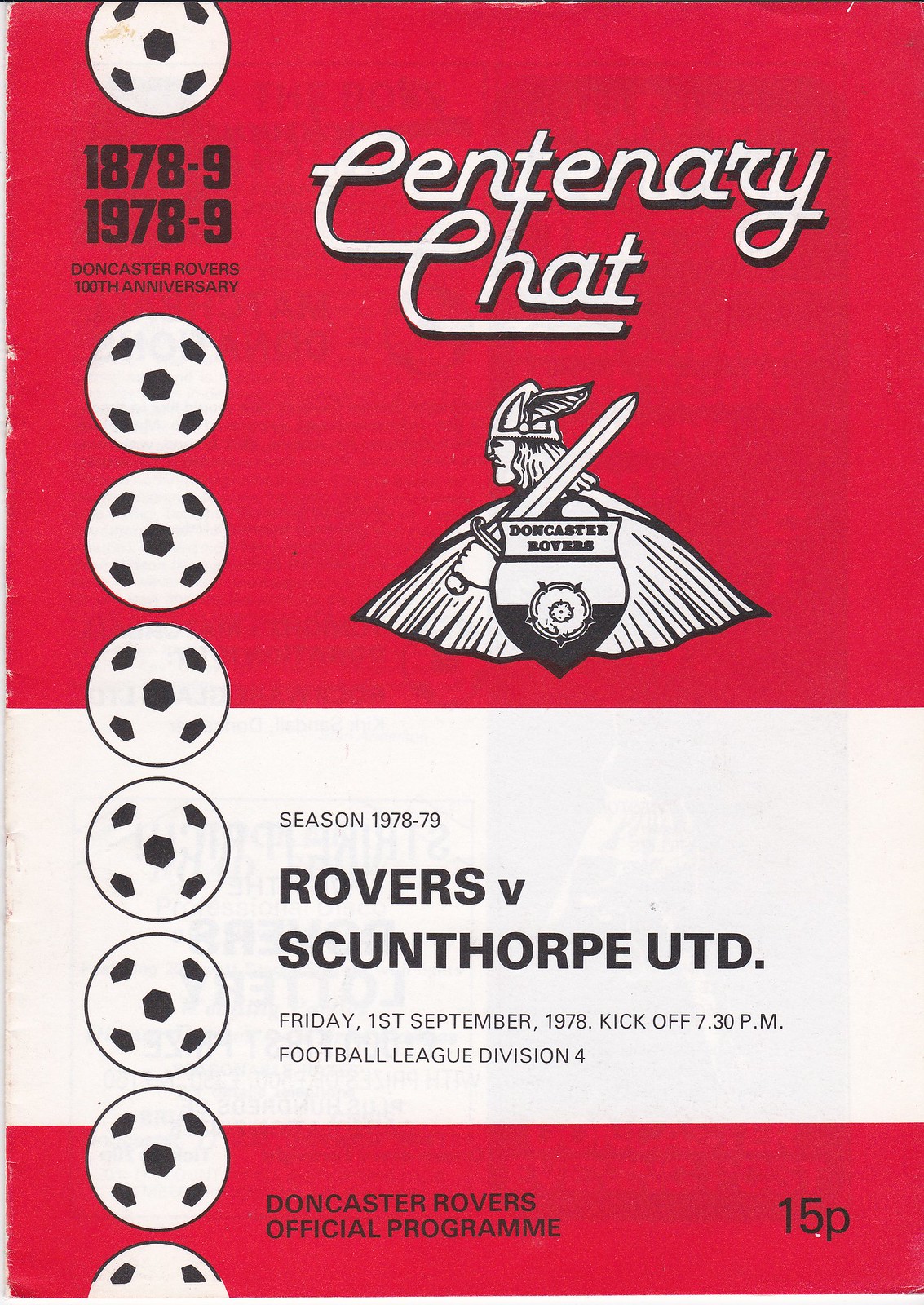The front cover of this soccer program, celebrating Doncaster Rovers' 100th anniversary, is primarily red with a white rectangular section in the middle. The top left corner features the dates "1878-9" and "1978-9" in black font along with "Doncaster Rovers' 100th Anniversary" against the red background. A column of illustrated black-and-white soccer balls runs vertically along the left edge. Centered in stylized white cursive script is the title "Centenary Chat." Below that, a logo displays a Viking in profile, wearing a winged helmet and holding a sword, with a shield emblazoned with "Doncaster Rovers" in front. The white middle section contains the matchup details in black font: "Season 1978-79, Rovers vs. Scunthorpe UTD, Friday, 1st September 1978, kickoff 7.30 p.m., Football League Division IV." The cover concludes with a smaller red strip at the bottom, stating "Doncaster Rovers official program, 15P" in black text.